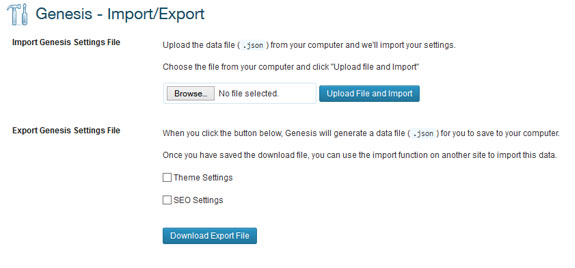Screenshot of Import/Export Interface for Genesis

This screenshot displays an import/export interface for an application titled "Genesis-Import-Export". The title, situated in the top left corner, is formatted as "Genesis-Import-Export" with a forward slash separating the words "import" and "export".

The main functionality of this page appears to be file management, allowing users to upload and download data files. Immediately below the title is a brief description guiding the user: "Upload the data file from your computer and we'll import your settings. Choose the file from your computer and click upload file and import." 

In the central area of the page, there's a section where users can browse and select a file. A small browse button is located here, accompanied by a message indicating that no file has been selected. To the right of this browse area is a blue button labeled "Upload File and Import", intended for uploading the chosen file.

At the bottom of the page, further instructions are provided: "When you click the button below, Genesis will generate a data file for you to save on your computer. Once you have saved the download file, you can use the import function on another site to import this data." This additional description clarifies the page's functionality, detailing the file export process.

Overall, the interface is designed for users to either upload a data file to import settings or download a data file for use on another site, facilitating data transfer within the Genesis application ecosystem.